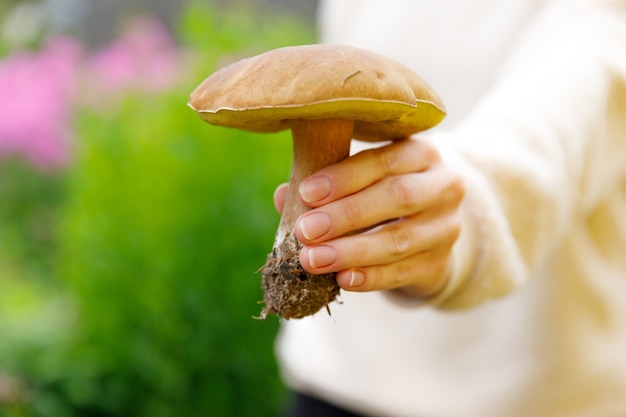In this photograph, a person's left hand, likely a woman's given the Caucasian skin tone and the length of the nails with white tips, is centrally positioned holding a freshly picked, large mushroom. The mushroom has a tan-colored cap with a much lighter, almost white, stem, and you can see dark brown dirt still clinging to its roots, emphasizing its recent extraction from the ground. The hand and mushroom are situated against a background that is slightly blurred but shows green vegetation and pink flowers, suggesting the setting is outdoors, likely during the day. The person’s arm is clad in a white long-sleeved sweater, adding a textured contrast to the earthiness of the mushroom and the natural surroundings. The rectangular, horizontal frame focuses on the hand and mushroom while capturing the serene, plant-filled environs, giving the image a tranquil, organic ambiance.